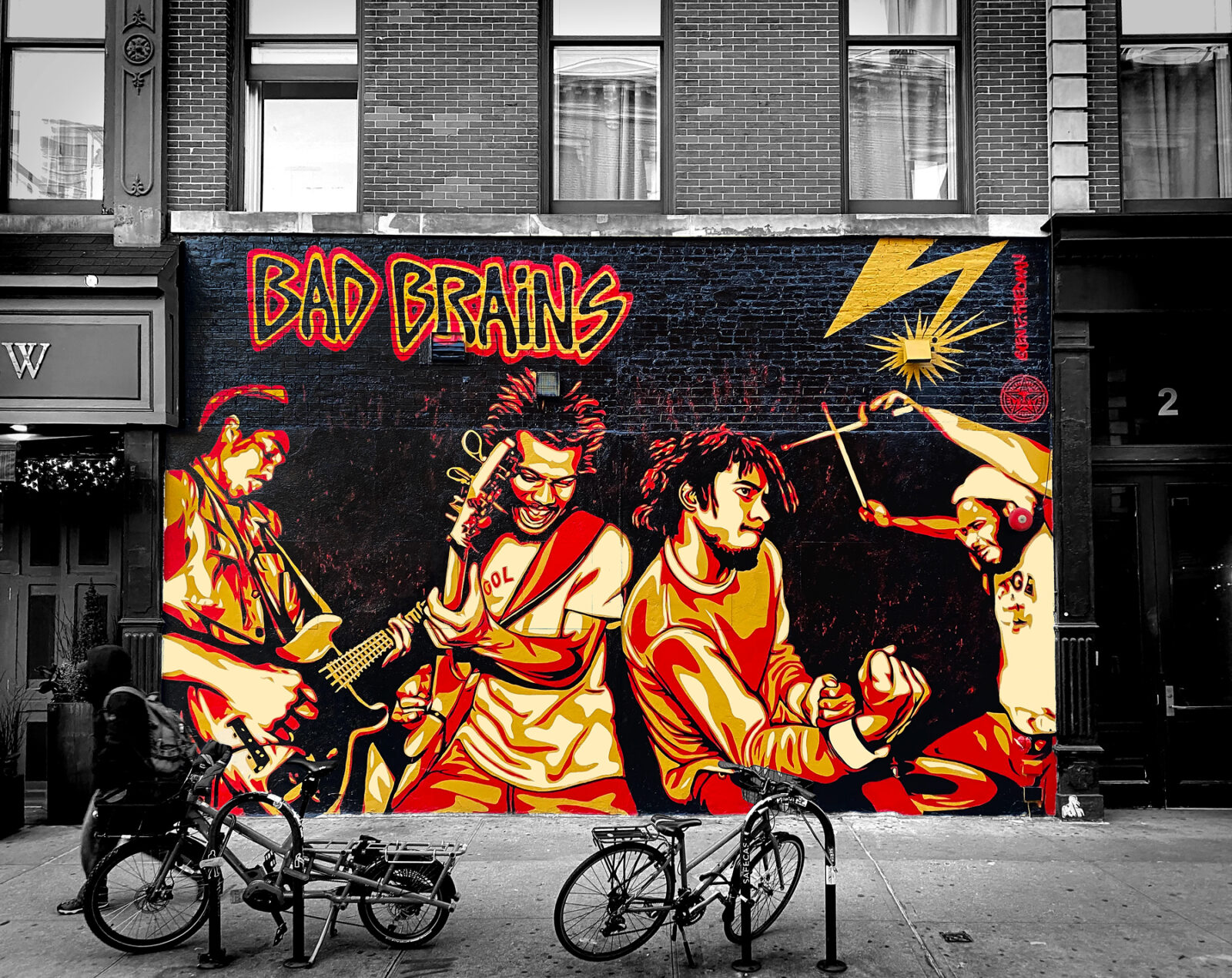The photograph captures a vivid urban artwork displayed on the side of a brick building. The scene is predominantly rendered in black and white, but the centerpiece, a vibrant mural, commands attention with its bold colors. The mural, professionally executed and likely commissioned, features the African-American punk band Bad Brains. The band's name is prominently displayed at the top in black letters, bordered first by yellow and then by red, adding to the visual impact.

Depicted in the mural are four musicians energetically engaging with their instruments: two playing guitars, one playing the drums, and another seemingly throwing up drumsticks. One of the musicians strikes a dynamic pose, his fist pumped in a gesture of positive aggression. In front of the mural, the street scene includes two bicycles locked to metal racks and a pedestrian walking along the sidewalk, adding a layer of urban life to the composition. The contrast between the monochromatic background and the colorful mural highlights the artwork’s vivid details, making it pop with warm tones of yellow and red, enhancing its presence in the filtered photograph reminiscent of social media aesthetics. The setting is well-lit, further emphasizing the clear, sharp details of the image.